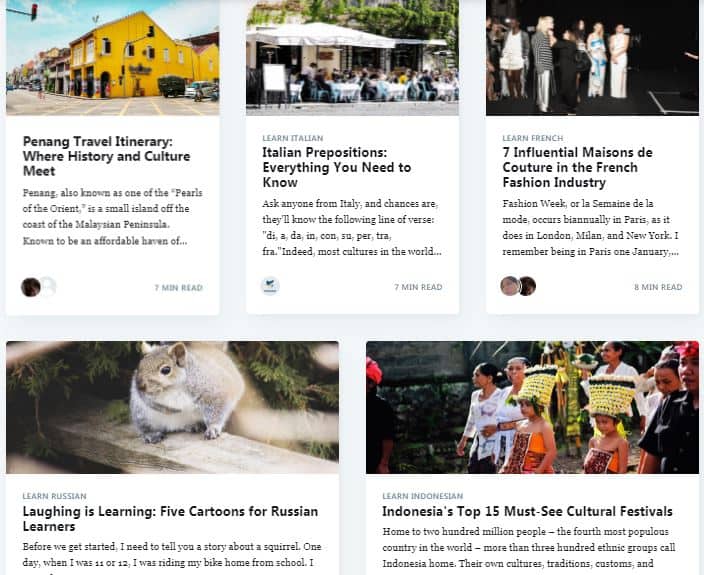**Detailed Caption for the Image:**

The image appears to be a collage of various articles from a news aggregate, each featuring distinct cultural and educational themes:

1. **Top Left Section:**
   - **Visual Description:** The top left section showcases an orange building amidst a cluster of red and brown buildings. The sky is a vivid cyan blue dotted with white clouds. Below the buildings lies a light gray parking lot that shows signs of wear, including white spots and fading. The scene includes several cars and people scattered on both the left and right sides.
   - **Textual Elements:** There is a white square containing bold black text that reads, "Penang Travel Itinerary: Where History and Culture Meet." Below, in normal black text, it introduces Penang, also referred to as one of the "Pearls of the Orient," a small island off the coast of the Malayan peninsula known for being an affordable haven. The excerpt is cut off with ellipses. Additionally, "7-minute read" is displayed in blue text at the lower right.

2. **Second Section:**
   - **Visual Description:** This section depicts people seated outside a cream-colored building with a white roof, adjacent to a black building.
   - **Textual Elements:** The heading "Learn Italian" appears in gray. Below that, in bold black text, is the title, "Italian Prepositions: Everything You Need to Know." The description begins with, "Ask anyone from Italy, and chances are they'll know the following prepositions: di, a, da, in, con, su, per, tra, fra." The passage ends with ellipses and mentions it’s a 7-minute read.

3. **Third Section:**
   - **Visual Description:** This section shows a group of people standing outside. On the right, two women are wearing dresses—one floral in blue and white, and the other in white. A man in a black and gray striped shirt with white pants stands next to a woman dressed entirely in black, who appears to be playful.
   - **Textual Elements:** It reads "Learn French" in gray. Beneath that, the bold black text states, "Seven Influential Maisons de Couture in the French Fashion Industry." The text continues to talk about fashion week, "La Semaine de la Mode," happening biannually in Paris, London, Milan, and New York. The sentence cuts off with ellipses.

4. **Fourth Section:**
   - **Visual Description:** A brown, gray, and white squirrel is positioned in the lower left corner.
   - **Textual Elements:** The section is titled "Learn Russian" in gray. In bold black text, it states "Laughing is Learning: Five Cartoons for Russian Learners." The narrative starts with, "Before we get started, I need to tell you a story about a squirrel. One day, when I was 11 or 12, I was riding my bike home from school," but the text is cut off.

5. **Last Section:**
   - **Visual Description:** The final section displays girls carrying wicker baskets atop their heads, colored yellow with a black stripe. They wear orange dresses adorned with maroon red and black floral patterns. Women clad in black and white, along with men in black, can be seen in the background.
   - **Textual Elements:** The heading "Learn Indonesian" appears in gray. The bold black text reads, "Indonesia's Top 15 Cultural Festivals." Below that, the normal black text begins to describe Indonesia, home to 200 million people (the fourth most populous country in the world) and more than 300 ethnic groups. The sentence is cut off mid-description.

This detailed visual and textual analysis of the image provides a comprehensive understanding of its content, blending cultural insights with educational themes across various languages and regions.